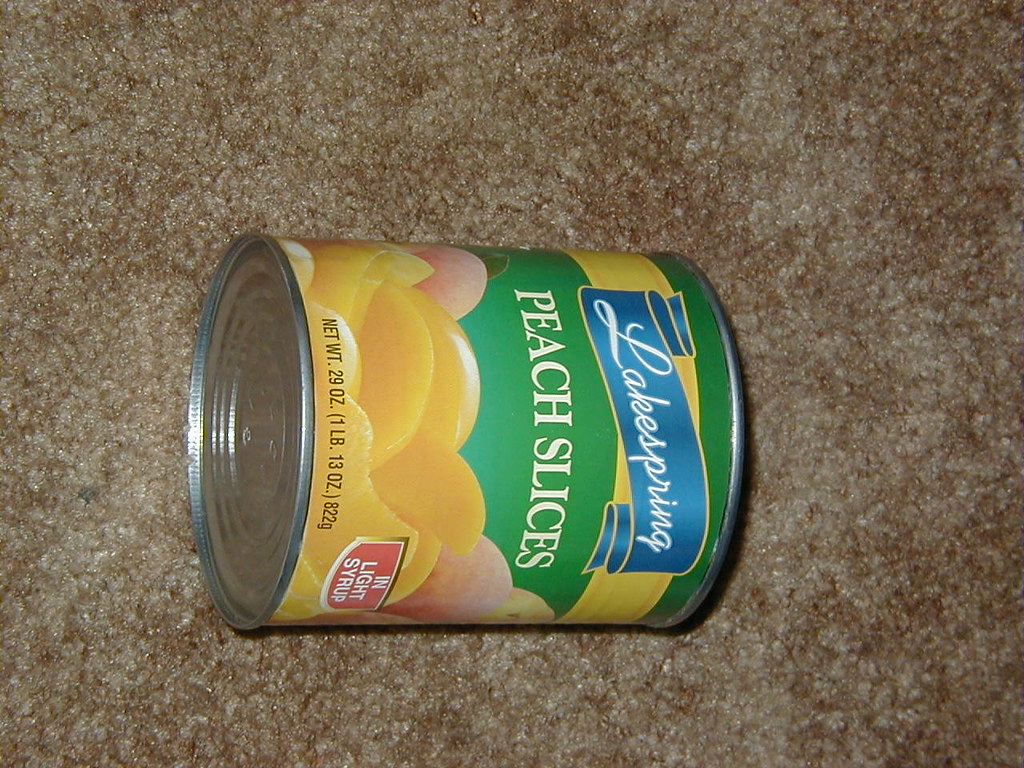This image depicts a can of Lake Spring peach slices in light syrup, with a net weight of 29 ounces (1 pound 13 ounces or 822 grams), lying sideways. The photograph is taken from a slightly top-down angle on a brown and light tan carpet. The can's label is detailed with a green section featuring the words "peach slices" in white. A yellow ribbon or ring accents the top of the green section, followed by a blue banner with the brand name "Lake Spring" written in cursive white text. The can's design includes images of whole and sliced golden peaches at the bottom. The contrasting golden peaches and vibrant labels make the product visually appealing, although there is a slight distortion on the right side of the can, giving it an odd look. The image composition prominently displays both the labeling and the bottom of the can.